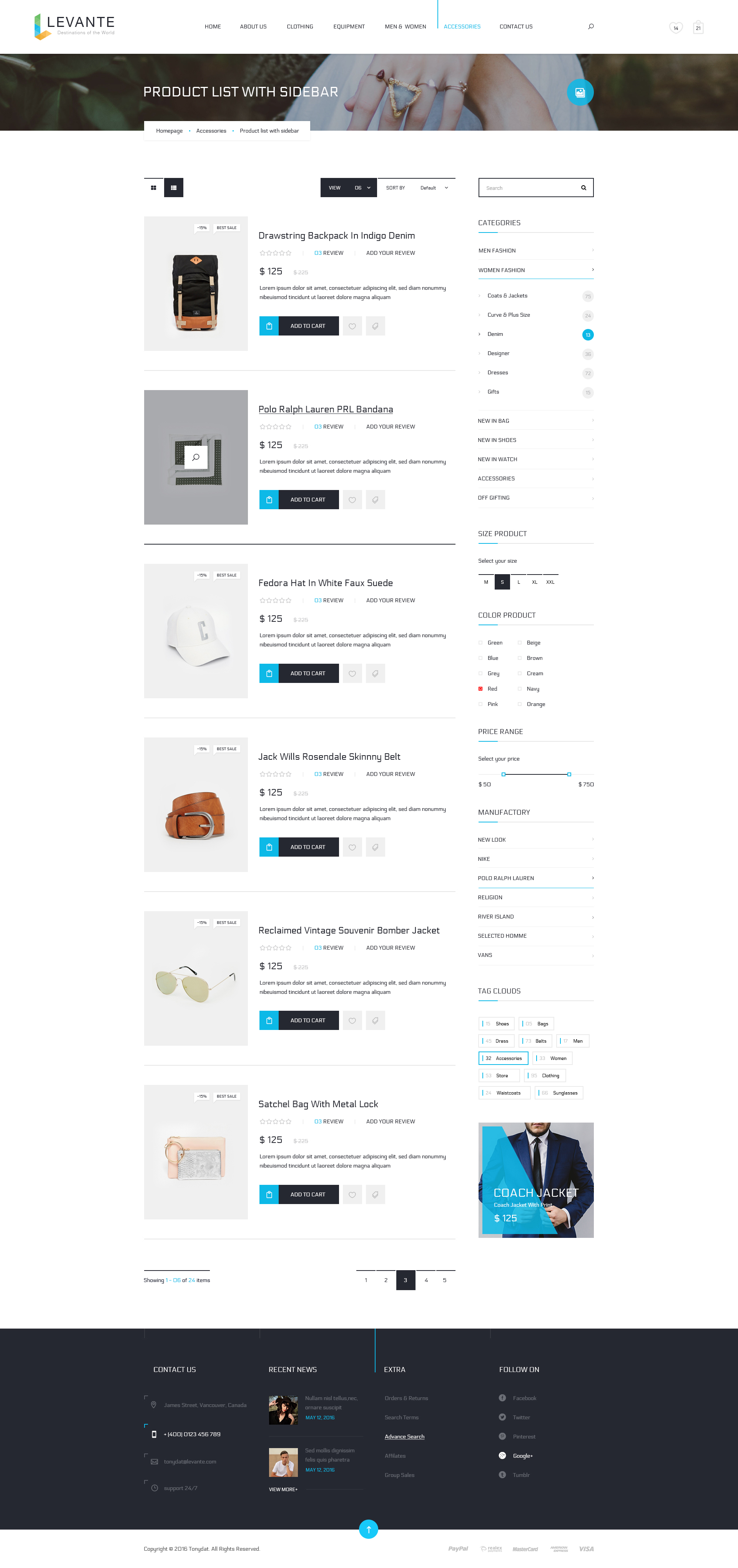In the image, which appears to be a snapshot of the Levante website, the branding is clearly visible in the top left corner. The Levante logo, featuring an "L" composed of blue and yellow segments, is prominently displayed. To the right of the logo, there are several category headers, though the text is quite small and slightly blurred. It seems to list categories such as "Perfume," "Units," "Watches," and possibly others.

Beneath the header, there's an image of a woman's hand, adorned with a ring on her middle finger. To the left of this image, the words "Product List with Sidebar" are visible, indicating the layout of the webpage. Progressing down the center of the page, multiple products are listed with accompanying images and prices:

1. **Drawstring Backpack in Indigo Denim** - Displayed to the left side with a price tag of $125.
2. **Polo Ralph Lauren DRL Bandana** - Listed below the backpack, also priced at $125.
3. **Fedora Hat in White Fox Suede** - Positioned centrally within the image, priced at $125.
4. **Jake Wills Rosemade Belt** - Displayed next with a listed price of $125.
5. **Reclaimed Vintage Souvenir Bomber Jacket** - Priced at $125 and listed below the belt.
6. **Satchel Bag with Metal Locks** - The final item, also priced at $125, located at the bottom of the product list.

Each product is showcased with a concise description and uniform pricing, providing a clear and structured view of the offerings on the Levante website.